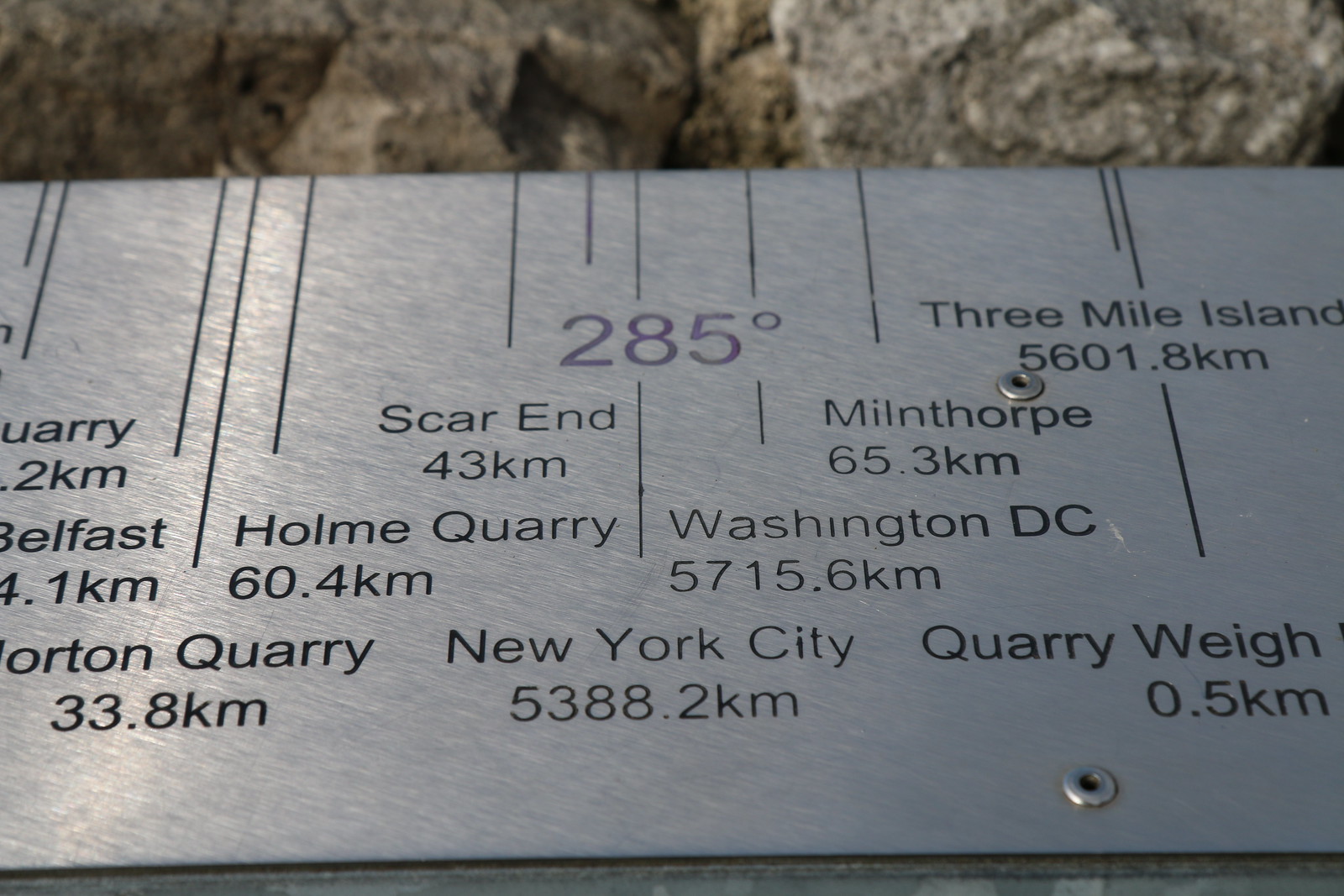The image displays a silver metal marker, mounted onto a rocky surface, with a slight angle making the bottom appear larger than the top. The marker, which resembles a ruler, features various vertical lines, black notches, numbers, and letters. It is securely screwed into place, visible against a background of grey boulders. The marker contains direction and distance information for several locations. Some are clearly readable: Norton Quarry at 33.8 km, Home Quarry at 60.4 km, Scar End at 43 km, and New York City at 5388.2 km. Other locations listed include Belfast at 4.1 km, Three Mile Island at 5601.8 km, Minthorpe at 65.3 km, Washington D.C. at 5715.6 km, and Quarry Way at 0.5 km. A central point marked as 285 degrees is prominently noted on the plaque, along with other locations arranged in a somewhat random manner.